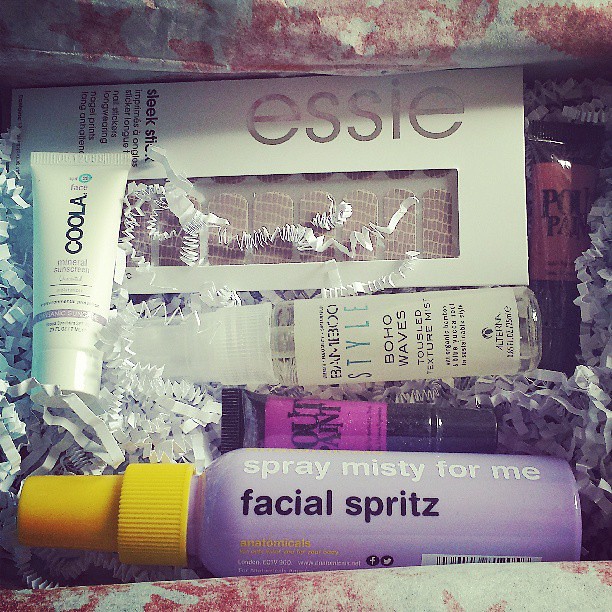The image showcases a content-rich toiletry subscription box set in pinkish-white tones with floral pink and white tissue paper, as well as shredded confetti paper. Prominently displayed is an assortment of beauty and skincare products, including an Essie Sleek Stick Nail Stickers box with visible snake skin nail stickers, positioned at an angle. Beside it, there's a white squeeze bottle labeled Coola, likely a mineral or organic sunscreen. Below that, a Bamboo Style Boho Waves Tussled Texture Mist spray bottle containing a clear liquid can be seen. The box also contains a purple bottle with a yellow lid labeled "Spray Misty for Me Facial Spritz" from Anatomicals. Additionally, there's a reddish and a black tube, with part of the label reading "POU," hinting at a lip color product. Each item is partially obscured by the decorative filler, adding an element of intrigue to the curated selection.